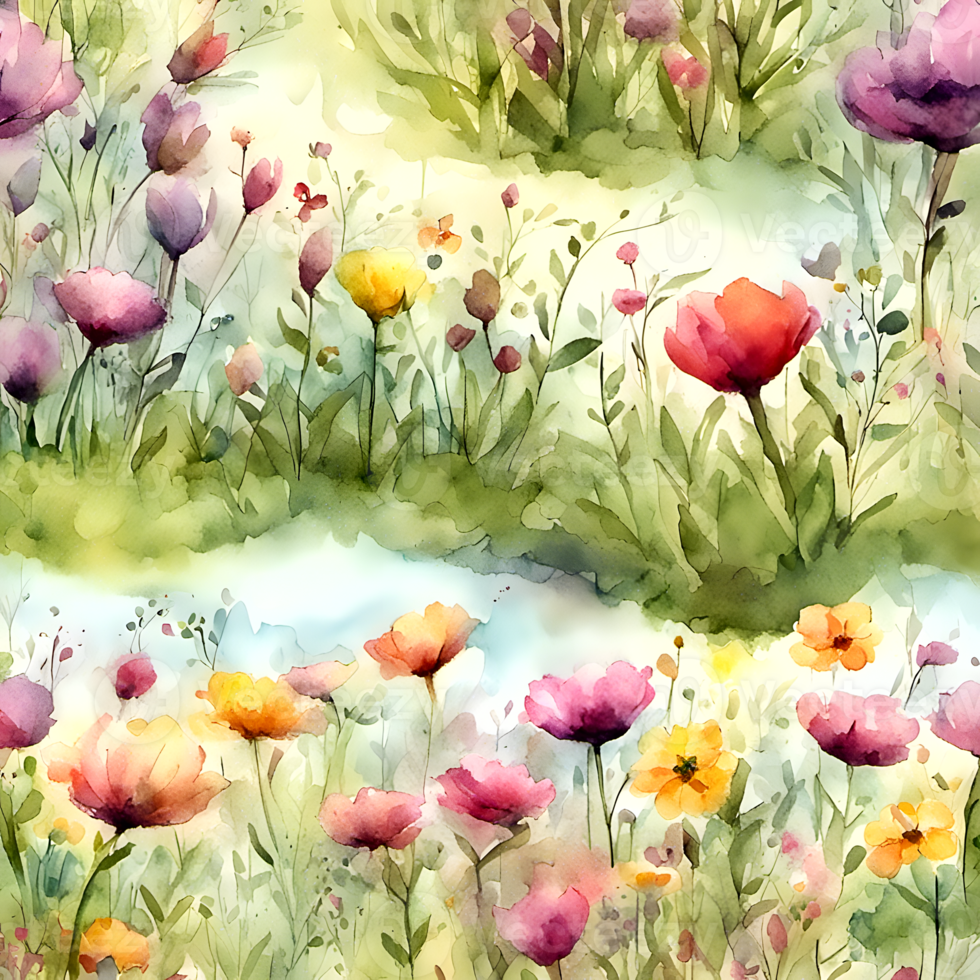The image appears to be an AI-generated watercolor painting depicting a vibrant garden scene from a slightly elevated, vertical perspective. The composition is rich with colorful flowers in various hues including red, orange, yellow, blue, pink, and purple, all of which are interspersed among lush green leaves and stems. These flowers are organized in three distinct rows that are separated by light tan earthen paths, providing a rustic and charming country meadow atmosphere. The foreground of the painting features primarily yellow and reddish-pink flowers, transitioning to violet and sparser yellow flowers in the middle row, with a mix of greenery and a prominent violet flower in the upper right corner. The delicate, rispy quality of the watercolor strokes adds to the illustration's ethereal and whimsical aesthetic, making it a captivating portrayal of a tranquil garden setting.